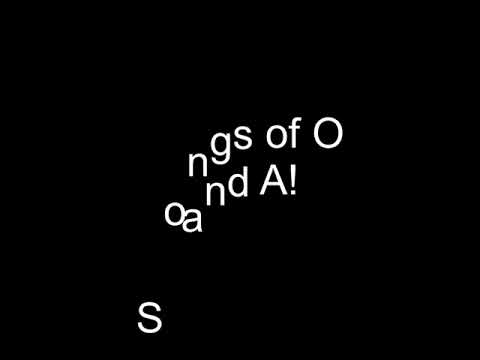The image is a black square with a unique arrangement of bold white text towards the center but slightly above the midpoint. The text reads "Songs of O and A!" in a wavy, flowing pattern. Specifically, "songs" starts horizontally with the letters S, O, and N, then dips down with the G and rises again with the S. The word "of" follows horizontally at the same level as the top of the previous S, while a large capital "O" is positioned further below. Continuing this undulating design, the words "and A!" follow a similar up-and-down wave, creating a dynamic and visual rhythm to the composition. The entire design emphasizes a playful yet structured placement of the text on a stark black background.